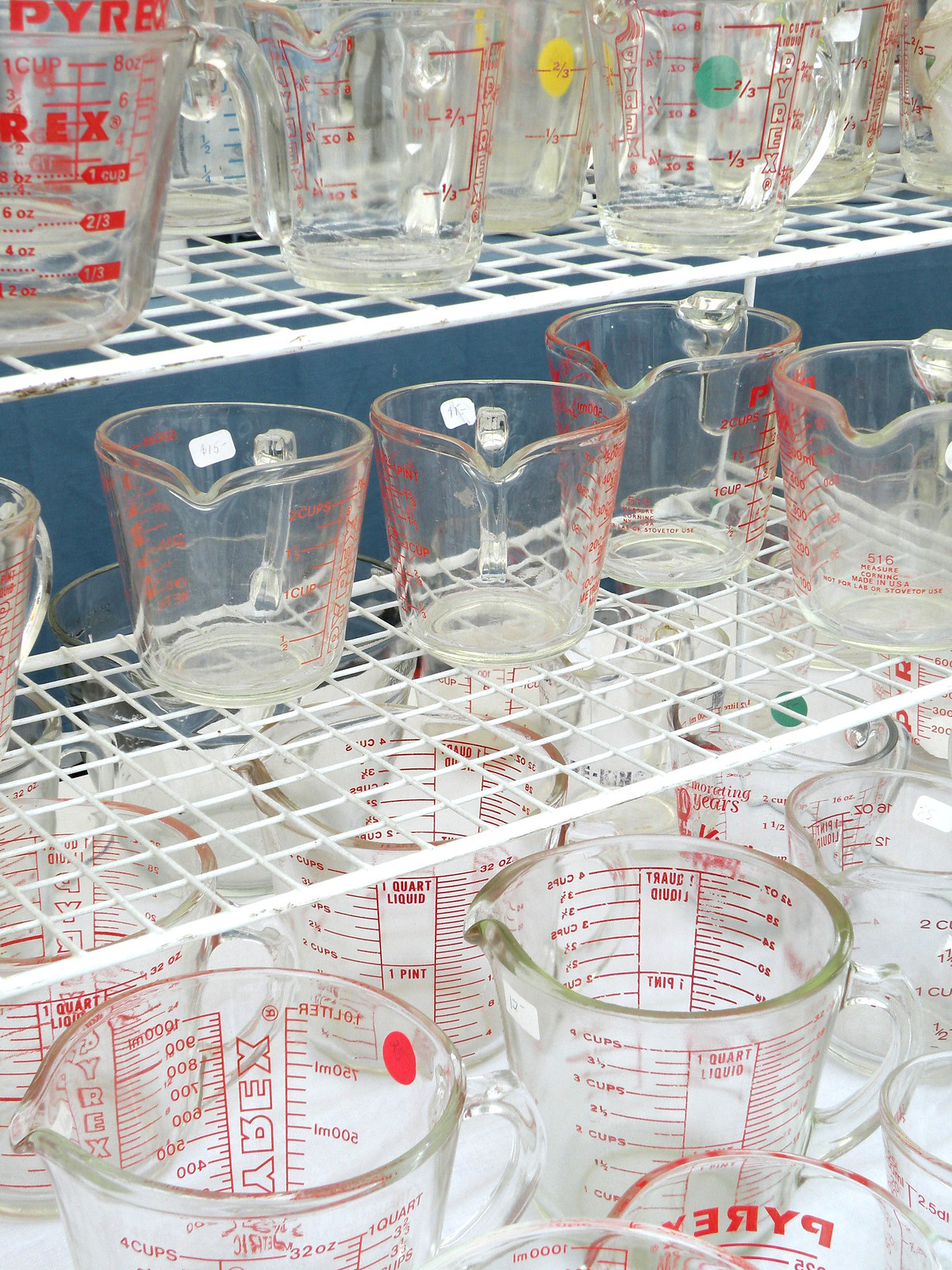This color photograph, likely taken inside a kitchen store or similar retail environment, captures three rows of white wire shelves lined with clear glass Pyrex measuring cups. Each measuring cup features distinctive red markings to indicate various measurements in both cups and ounces, as well as the brand name "Pyrex" prominently displayed in red. The measuring cups, which have spouts and handles, are organized neatly in rows on the shelves. The top shelf holds smaller measuring cups, each capable of holding up to one cup, with subdivisions for one-third, two-thirds, and one cup. The middle shelf presents medium-sized measuring cups, each capable of holding up to two cups, with markings for half-cup, one cup, one and a half cup, and two cups. The bottom shelf contains the largest measuring cups, each capable of holding up to four cups, with subdivisions for one, two, three, and four cups. Some measuring cups have white price stickers, while others have yellow, green, or red stickers, possibly indicating different prices or conditions. The blue riser supporting the middle shelf adds a contrasting pop of color. The organized display of Pyrex measuring cups suggests a well-stocked, indoor retail setting.